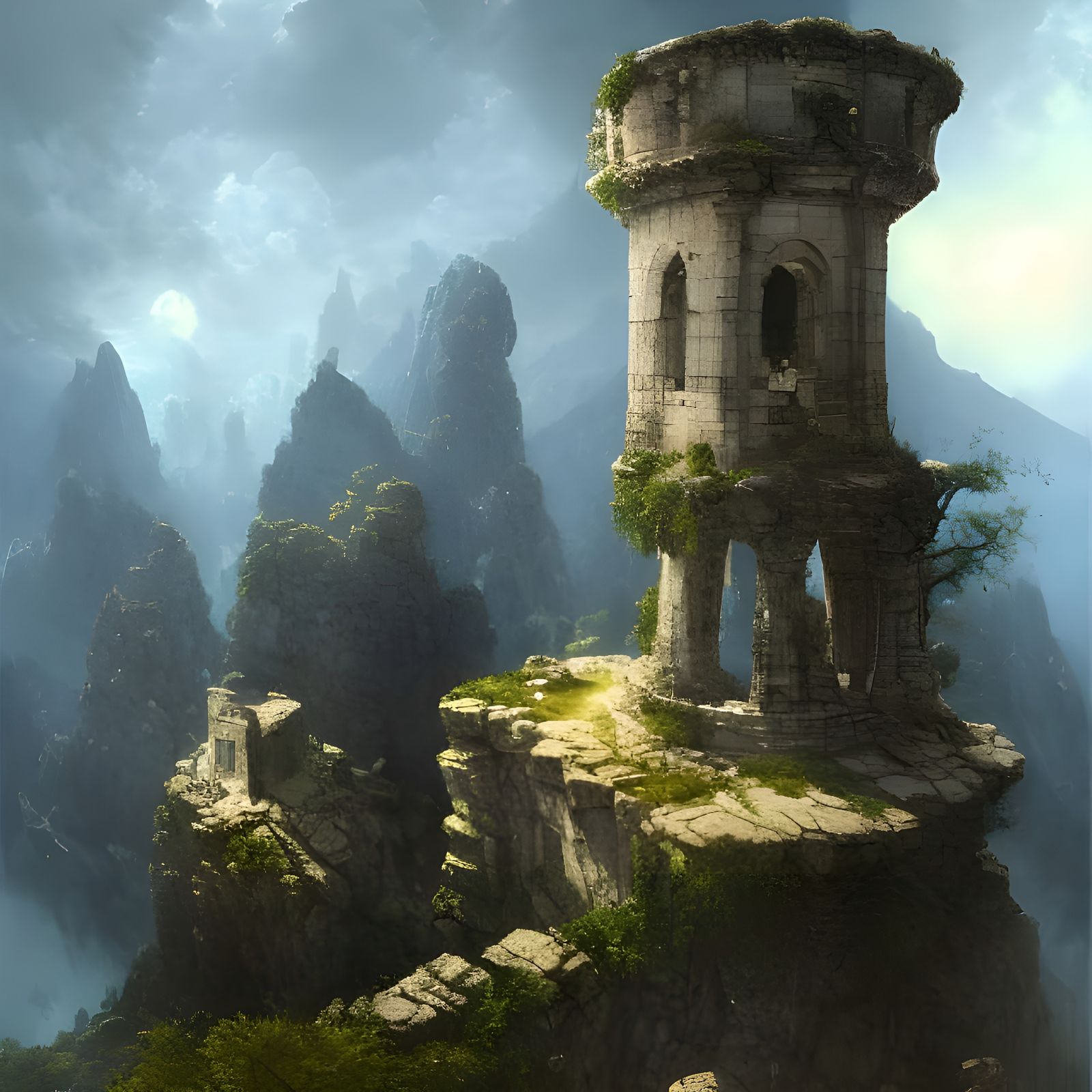The image depicts an artistic rendering of a deteriorating, cylindrical tower perched atop a distinct, pillar-like mountain. The tower, which is partially crumbling and overgrown with greenery, features four pillars supporting a second story and boasts tall, rounded windows—one of which may even contain a face. The scene includes additional rocky, column-like mountains scattered around, some adorned with small, stone structures, all in varying states of ruin. The remnants of disconnected stone paths hint at a network that once linked these mountains. In the foreground, a deteriorated path with only a few stones left suggests further disintegration. In the background, larger, pointed peaks resembling those found in karst landscapes, possibly influenced by Chinese topography, reach towards a cloudy sky, with a moon visible in the upper left corner. The scene, reminiscent of settings from "The Legend of Zelda: Breath of the Wild" or a fairy tale like Rapunzel, combines elements of hyper-realistic detail and fantasy to create a captivating, high-quality visual.